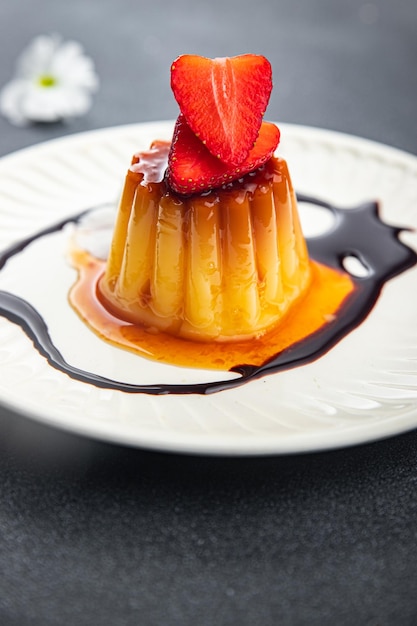This image features a delicious dessert that resembles either a cupcake or a scoop of ice cream, potentially molded from gelatin. The dessert is yellow in color and sits elegantly on a white plate. It is richly drenched in what appears to be a sweet caramel sauce, further accentuated by artistic drizzles of chocolate around it. Atop the dessert are two pieces of cut strawberries, likely halves from a single piece, meticulously placed to enhance its visual appeal. The white plate is positioned on a dark surface, adding contrast to the vibrant dessert. In the blurred background, a white flower with a greenish-yellow center, possibly a dandelion petal, adds a subtle touch of nature to the composition.